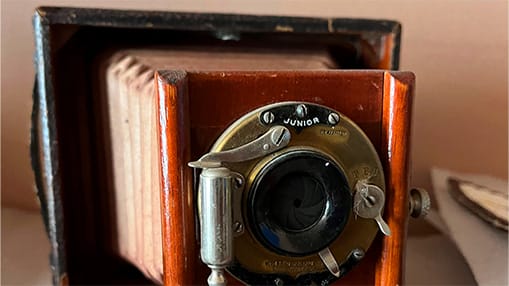This landscape-oriented photograph captures an intricately detailed vintage box camera. The camera features a distinctive black rectangular section at its rear, which is connected to a khaki-colored accordion-style bellows that extends towards the wooden front of the camera. The wooden front is of a reddish-brown hue and centrally positioned in the image. Prominently displayed on the wooden front is a brass circular plate adorned with various knobs and screws. Within this brass circle lies the lens apparatus, crafted from metal, which includes a black lens and a lens cover. An oval-shaped plate near the top of the circle bears the inscription "Junior," possibly denoting the brand or lens maker. The photograph focuses sharply on this front section, while the backdrop remains slightly blurred, hinting at the presence of indistinct shapes and a piece of paper.